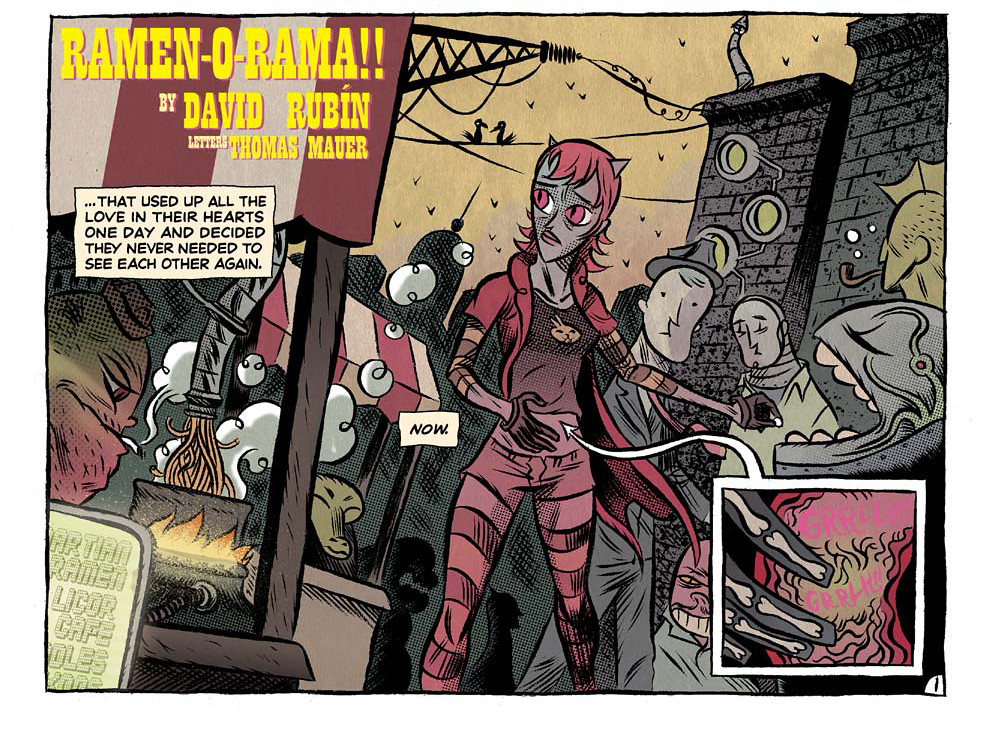The image appears to be a vibrant digital illustration in a comic book style, titled "Ramana Rama!!" by David Rubin, with lettering by Thomas Mauer. The yellow title text at the top is prominent. Below this, there's a central text box stating, "They used up all the love in their hearts one day and decided they never needed to see each other again." In the middle, a main female character with red hair, large red eyes, and sharp cat-like ears is featured. She wears striped high socks, a striped shirt, and shorts. Emphasizing a blend of the fantastical and the mundane, an arrow from her stomach leads to an X-ray square showing her fingers over her stomach, possibly indicating hunger – accentuated with the word "now" in another text box.

Surrounding her are various market scenes with a carnival-like atmosphere. To the left, stalls with red and white canopies display a fire and stove where a round-headed character looks down at a pan while smoking a cigarette. Further left is another booth with fire, contributing to a lively marketplace ambiance. The background is detailed with brick buildings, wires, and metal structures, establishing the setting. Additional characters and creatures populate the scene: a rounded creature with its eyes closed and mouth open is present near the main character, alongside other human and animal figures interacting in the market. The colors range broadly from reds, oranges, and blacks to light greens, yellows, and whites, enriching the illustration’s dynamic and bustling feel. Birds perched on a power line above add to the depth and busy nature of the scene.